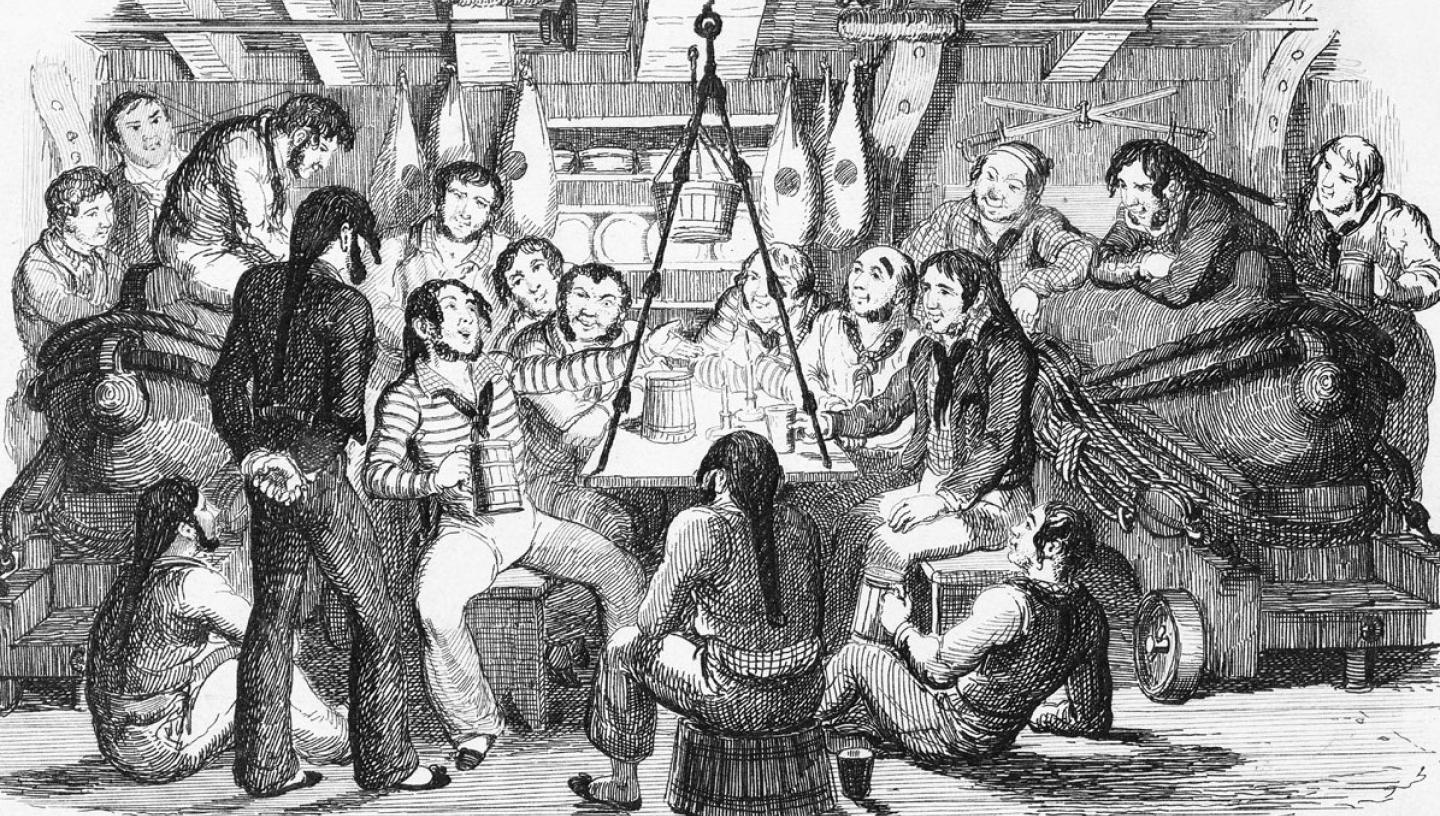This is an intricate, horizontal pen sketch illustrating a group of men, possibly pirates or sailors, gathered below deck on a ship. The aged, black-ink drawing features a cluttered space, with food and baskets hanging from the wooden walls and ceiling. At the center, a table is surrounded by men seated on benches, while others sit on cannons with wooden wheels, upturned buckets, and the floor. One dominant figure, dressed in a striped shirt with a dark tie, stands at the head of the table, arms extended and holding a beer stein, as if delivering an animated speech. All eyes are fixed on him. Scattered among these men are various structures, including an A-frame supporting a pot or bucket. The scene is bustling, almost convivial, as the men engage in what seems to be an important discussion or meeting, with some standing and hovering around, adding to the lively atmosphere of a bar-like setting aboard an old ship.